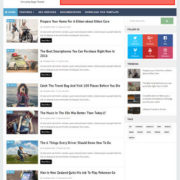The image presents a slightly out-of-focus grid-like structure consisting of six horizontal rows. Each row appears to contain articles, although the contents are difficult to discern due to the blur. The top of the image is marked by a prominent red bar. Below this bar are six colored squares: two in blue, two in red, one in dark blue, and one in pink. Interspersed among these squares, there are additional articles accompanied by some text, which remains unclear. The background of the image is predominantly white, with a few light blue squares scattered throughout. The overall composition suggests a webpage or a digital interface with categorized content, albeit obscured by the lack of clarity.